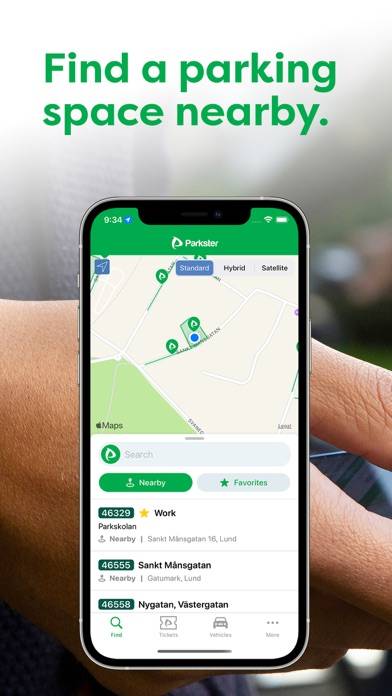The image showcases a webpage with the title "Parkster." Prominently displayed in large green letters is the phrase "Find a parking space nearby." The background of the image is blurred, but it reveals a hand holding a smartphone. However, the grip obfuscates the screen slightly—the back of the hand and fingers are visible, while the phone's display is partially hidden.

At the top of the phone's screen, "Parkster" is clearly visible. The status bar shows it is 9:34 AM. Below this, there is a map with green indicators, likely marking available parking spaces. Directly beneath the map, a search bar labeled "Nearby" in green can be seen. This implies that users can find parking locations in close proximity. The map also includes several green pins that probably represent parking spots. 

Further down, the interface presents options labeled "Favorites" with gray text detailed in green. The list includes various names and numbers, which appear to be location names and their respective distances. For example, "Pakistan Crack of Stone Stolen Park" and "Sankrit Men Got Tan" are mentioned, although these names might be garbled.

At the bottom of the smartphone's screen, there are different icons and a distinct black bar, likely part of the navigation menu.

Overall, the webpage and the smartphone display aim to assist users in efficiently finding nearby parking spaces through a visually simple yet informative interface.